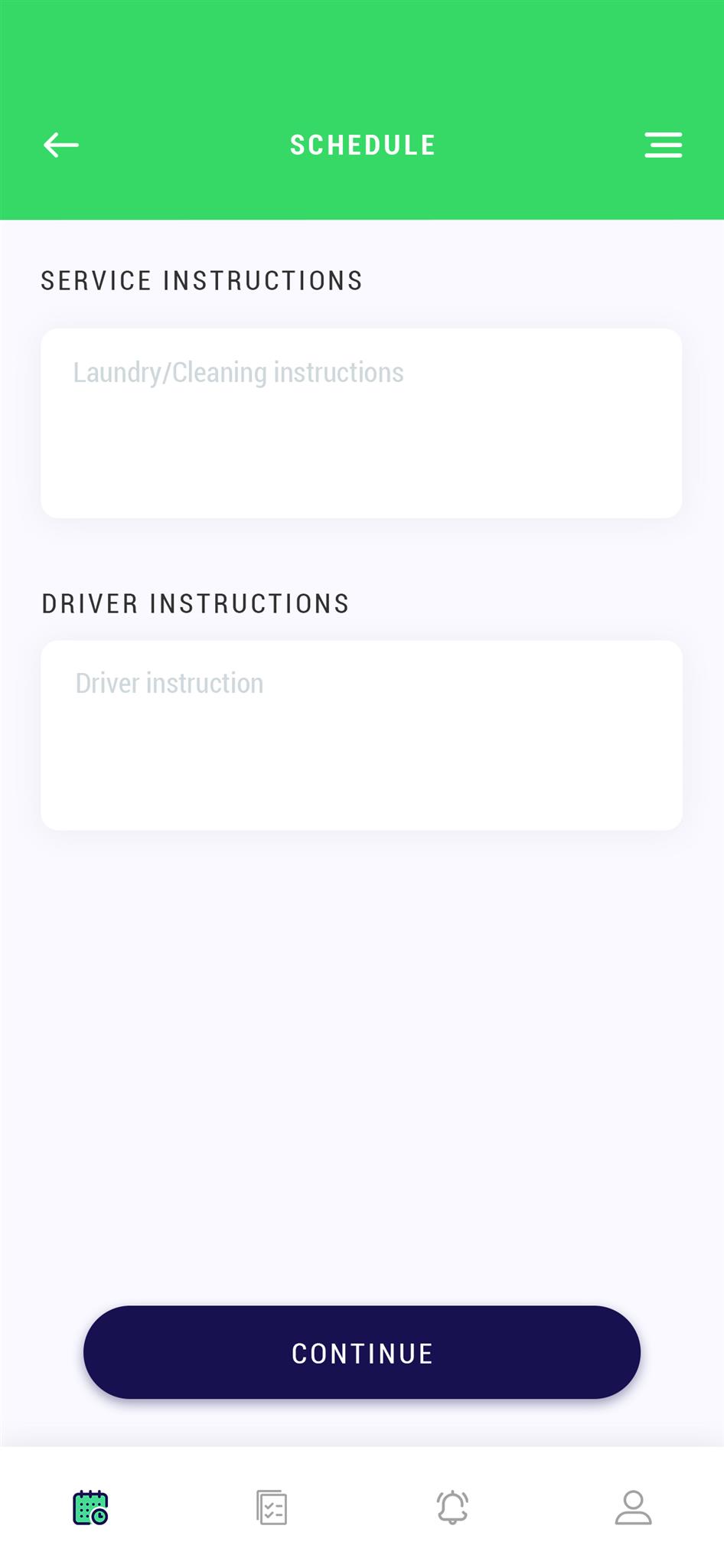The image depicts a mobile phone screen displaying what appears to be a scheduling application interface. At the very top of the screen, there's a back arrow located on the left and a three-line menu icon on the right. Centrally positioned in a green rectangular banner is the word "Schedule." 

Below this banner, the interface transitions to a black-and-white theme displaying various sections. The first section is titled "Service Instructions," which is further subdivided into "Laundry/Cleaning Instructions" and "Driver Instructions." There is an editable field provided for users to write specific driver instructions.

Further down, a blue button is present for users to click and continue to the next step. At the bottom of the screen, there is a navigational bar with multiple icons: a calendar icon, a text icon, an alarm bell icon, and a person icon. The calendar icon is highlighted in green, indicating the current selection is a calendar entry rather than a text note, alarm, or personal contact. The other icons are not highlighted, suggesting they are not in use in the current context.